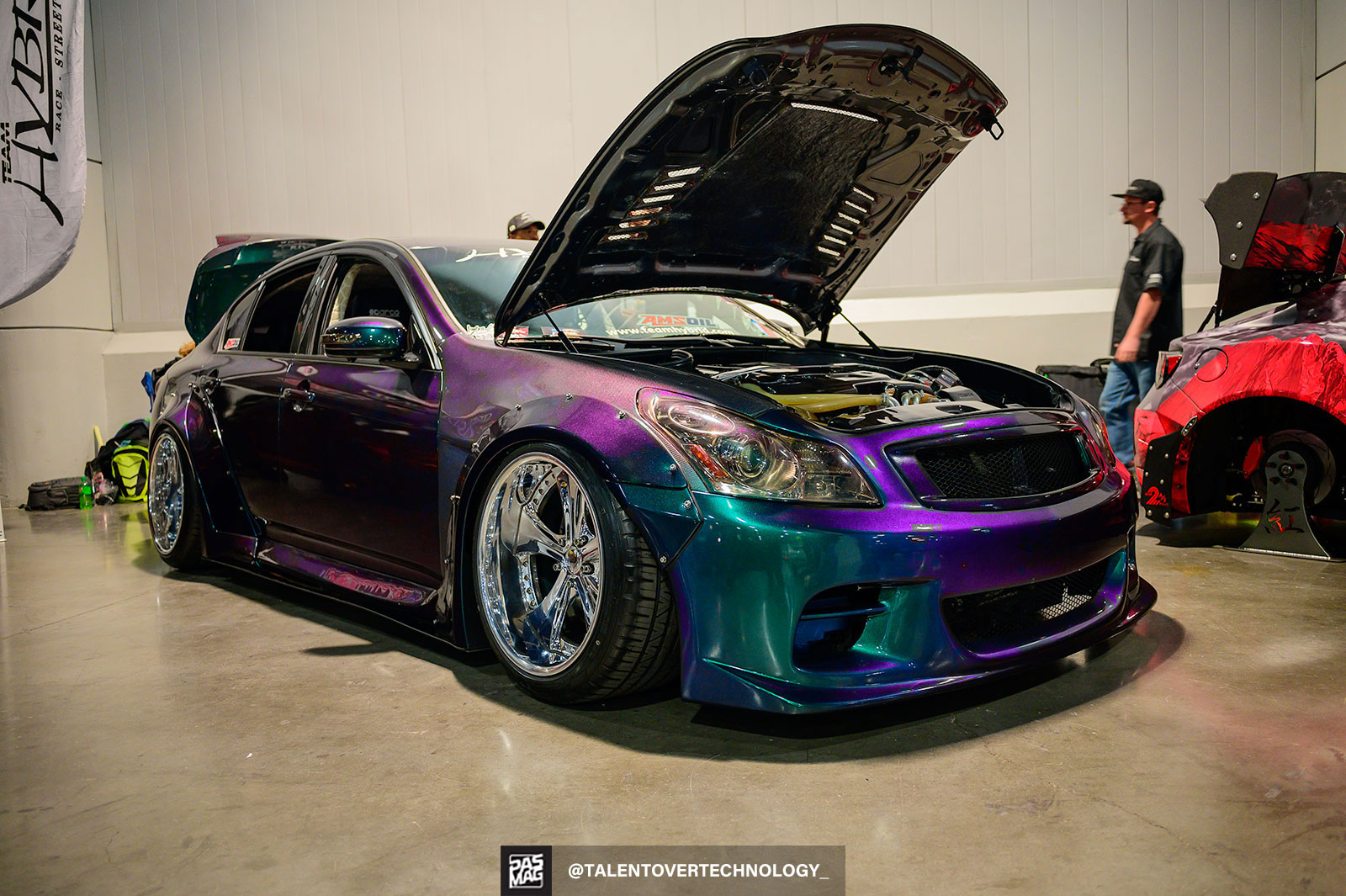The image captures a pristine garage or car showroom featuring a striking sports car as the focal point. The sports car boasts a unique pearlescent paint job that shifts between purple and aquamarine, giving it a vibrant, multi-hued appearance. This sleek vehicle is brand new with its hood and boot open, showcasing its inner mechanics. The windshield bears the AMS Oil logo and the website www.teamhybrid.com, hinting at a high-performance modification.

Two men in baseball caps are attentively inspecting different parts of the car, indicating a level of interest and expertise. Another car, covered in cloth and seemingly missing its wheels, is positioned to the right, further suggesting that the setting might be a specialized auto shop or exhibition space.

The clean, spacious environment features a smooth, brown, almost marble-like floor and white walls, contributing to a polished, sophisticated ambiance. A logo or branding statement at the bottom reads "Talent Over Technology," reinforcing the meticulous craftsmanship and ingenuity involved in these vehicles.